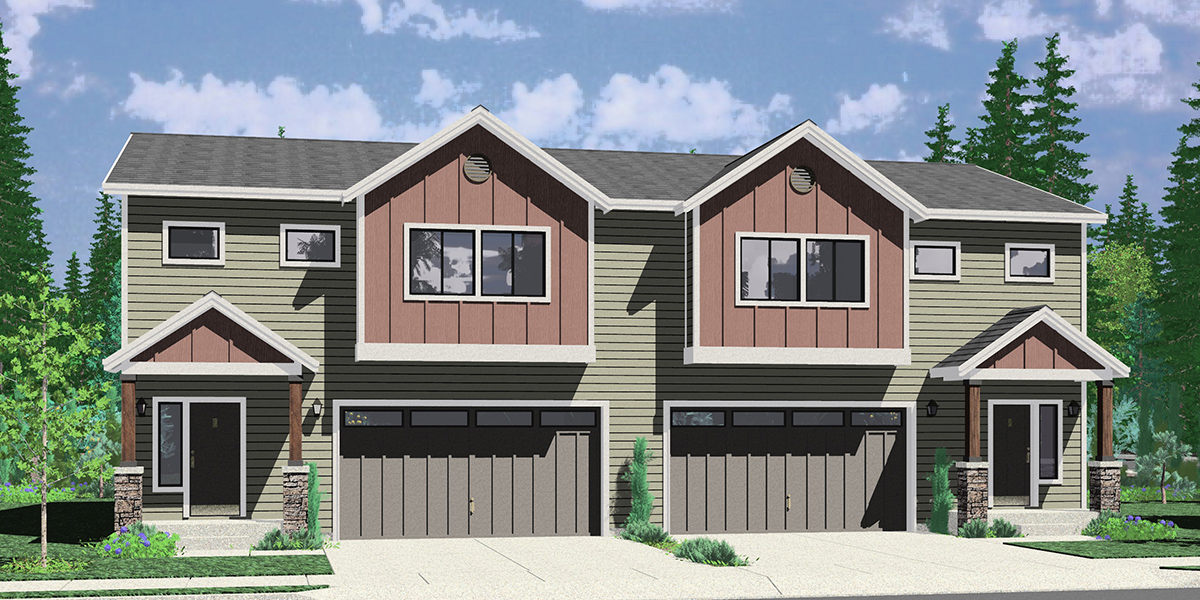This is a highly detailed architectural rendering of a duplex, showcasing two connected townhouses with crisp modern design elements. Both homes feature two stories with green vinyl siding on the majority of the exterior, complemented by light brown sections in the upper story and above the protruding frame areas. Each home has distinctive triangular peaked entrances supported by pillars that are stone at the base and transition to wood higher up.

The duplex presents symmetrical design where each side mirrors the other. Both townhouses have dark brown doors located at their respective ends, which are framed by covered porches supported by stone and wood pillars. The upper stories include large windows that match those found beneath in both green and brown sections. The peaked sections of the upper floor feature a circular design element at the apex.

The lower level of each townhouse includes a sizable dark gray garage door with an even pattern line running horizontally across. The duplex is topped with a dark gray tar roof and accented with maroon-rust and white trim. The foreground shows a paved concrete driveway leading to the garages, while the background is filled with tall trees and a partly cloudy sky. A smaller tree is planted to the left of the duplex, adding to the greenery in the scene. Overall, the architectural detail and landscape suggest a balanced combination of functionality and aesthetic appeal.